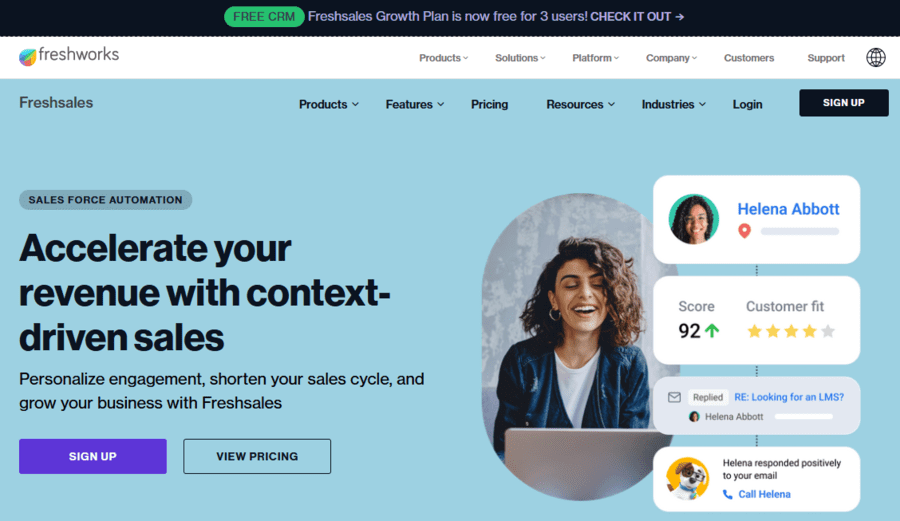This screenshot image is from the Freshworks website. At the very top, there is a black banner announcing that the "Free CRM Freshsales Growth Plan is now free for three users." Accompanying this text is an arrow pointing to the right.

Below this, there is a white banner containing text and various clickable tabs for navigation. The tabs available are:
- **Products** (with an arrow pointing downwards)
- **Solutions**
- **Platform**
- **Company**
- **Customers**
- **Support**

Directly beneath this white banner, the main body of the webpage has a light blue background. On the left-hand side of the top section, within a black box, the text reads "Freshsales." Adjacent to this, there are additional tabs:
- **Products**
- **Features**
- **Pricing**
- **Resources**
- **Industries**
- **Login**
And prominently featured in a black banner, there is a "Sign Up" button.

Under this navigation area, large text states "Salesforce Automation," followed by the phrase "Accelerate your revenue with context-driven sales." Further down, the text highlights key benefits: "Personalized engagement, shorten your sales cycle, and grow your business with Freshsales." 

Lastly, there are options to "Sign Up" and "View Pricing."

To the left of these textual descriptions, there is an image (not fully described in the provided text).